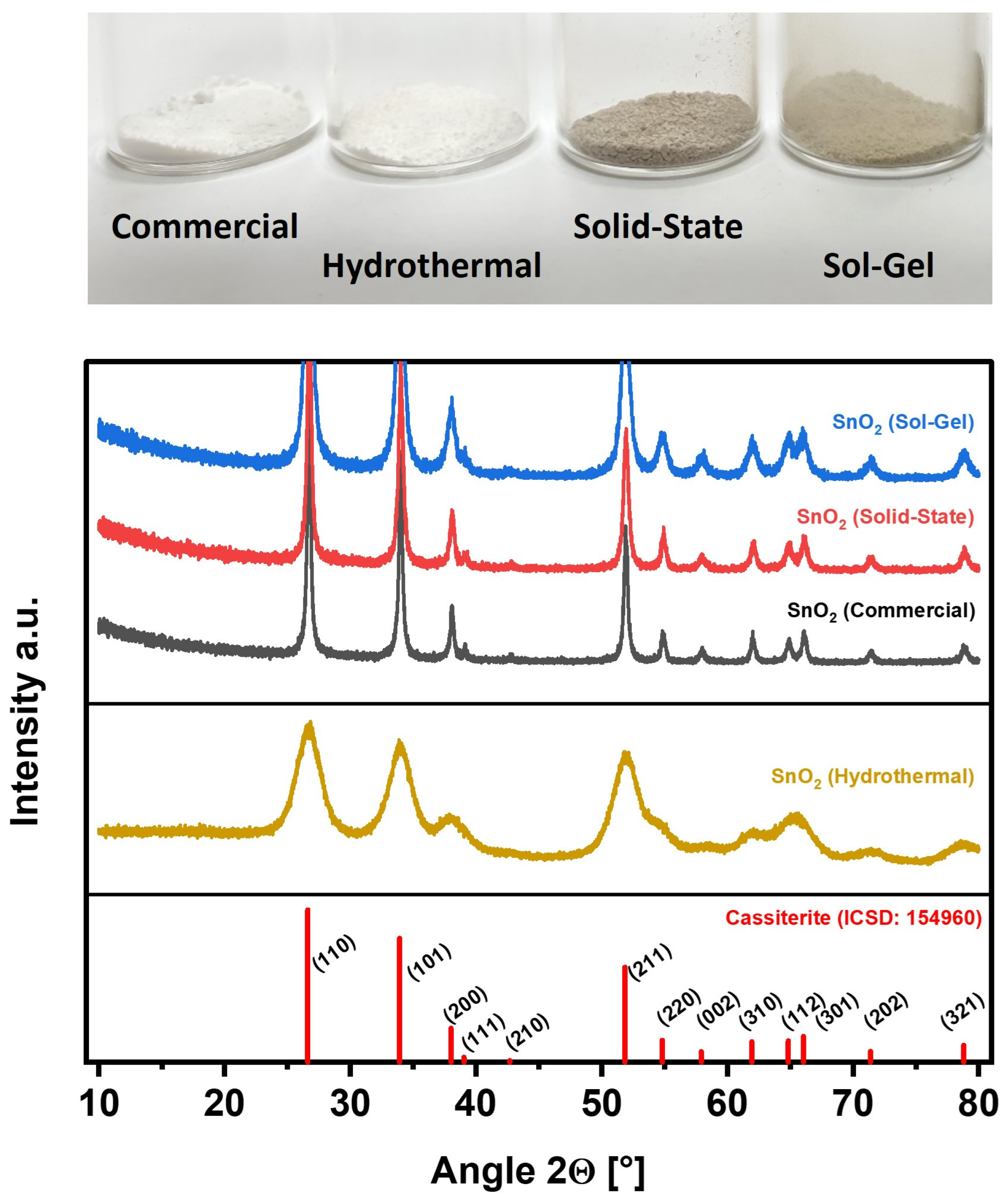The image displayed is oriented in portrait layout and is divided into two primary sections. At the top, against a gray background, there are four glass jars, each containing a small amount of a powdery substance, just covering the bottom. From left to right, these jars are labeled 'commercial,' 'hydrothermal,' 'solid state,' and 'sol-gel.' The first two powders are white, while the latter two are various shades of gray.

Beneath the jars is a graph divided into two rectangles, forming a square. The y-axis of the graph is labeled 'Intensity (a.u.),' and the x-axis is marked 'Angle (degrees)' ranging from 10 to 80. The upper rectangle features a multi-line graph with blue, red, and black lines, where blue peaks are highest, red peaks mid-level, and black peaks are the lowest. The lines represent different SNO (tin oxide) synthesis methods: sol-gel (blue), solid state (red), commercial (black), and hydrothermal (additional details from the first description).

The bottom rectangle contains a line graph in yellow, labeled 'cassiterite ICSD: 154960,' characterized by various lengths of lines indicating specific values. The graph's overall arrangement depicts a detailed comparison of the powder samples with respect to their intensity versus angle measurements.